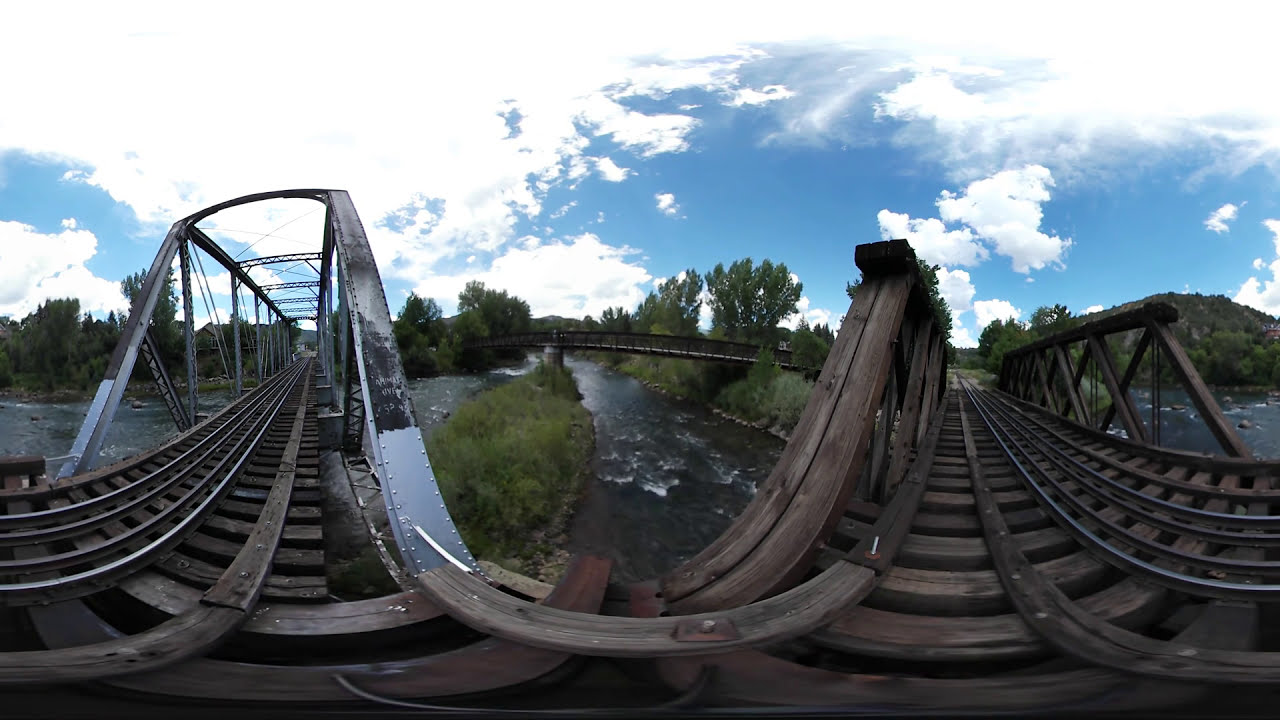This panoramic photograph depicts a pair of weathered train tracks running over a bridge that spans a murky river. The train tracks, appearing dilapidated and likely out of use, are divided by the water, with one set on the left and the other on the right, wrapping around the central point of the image. The tracks feature rusted, silvery-black metal support beams and failing wooden railings, highlighting their neglected state. The scene is set against the backdrop of a bright turquoise sky, with puffy white clouds scattered above. Surrounding the river are tall bushes and grasses, with lush green trees visible in the distance, enhancing the picturesque yet melancholic atmosphere of decay.